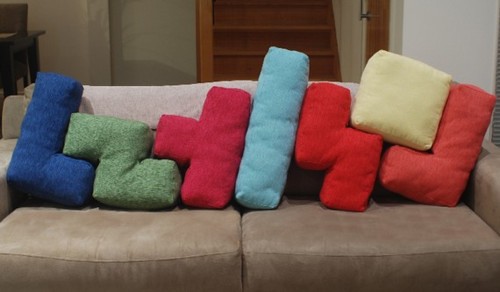The photograph captures a beautifully arranged living space adorned with a light brown love seat that dominates the lower two-thirds of the image. Against a backdrop of white cream-painted walls and a wooden staircase in the far background, the love seat is strikingly decorated with an assortment of vibrantly colored pillows, each shaped like different Tetris blocks. There is a navy blue L-shaped pillow, a green zigzag, a mellow pink-red T-shape, a light sky blue straight block, a bright red Z-shape, a yellow square, and an orangey-red standard pillow with a small white pillow placed on top. These uniquely shaped and colored pillows, suggestive of geometric forms from the game Tetris, create an eye-catching and unusual visual display that adds both aesthetic appeal and a playful touch to the setting.